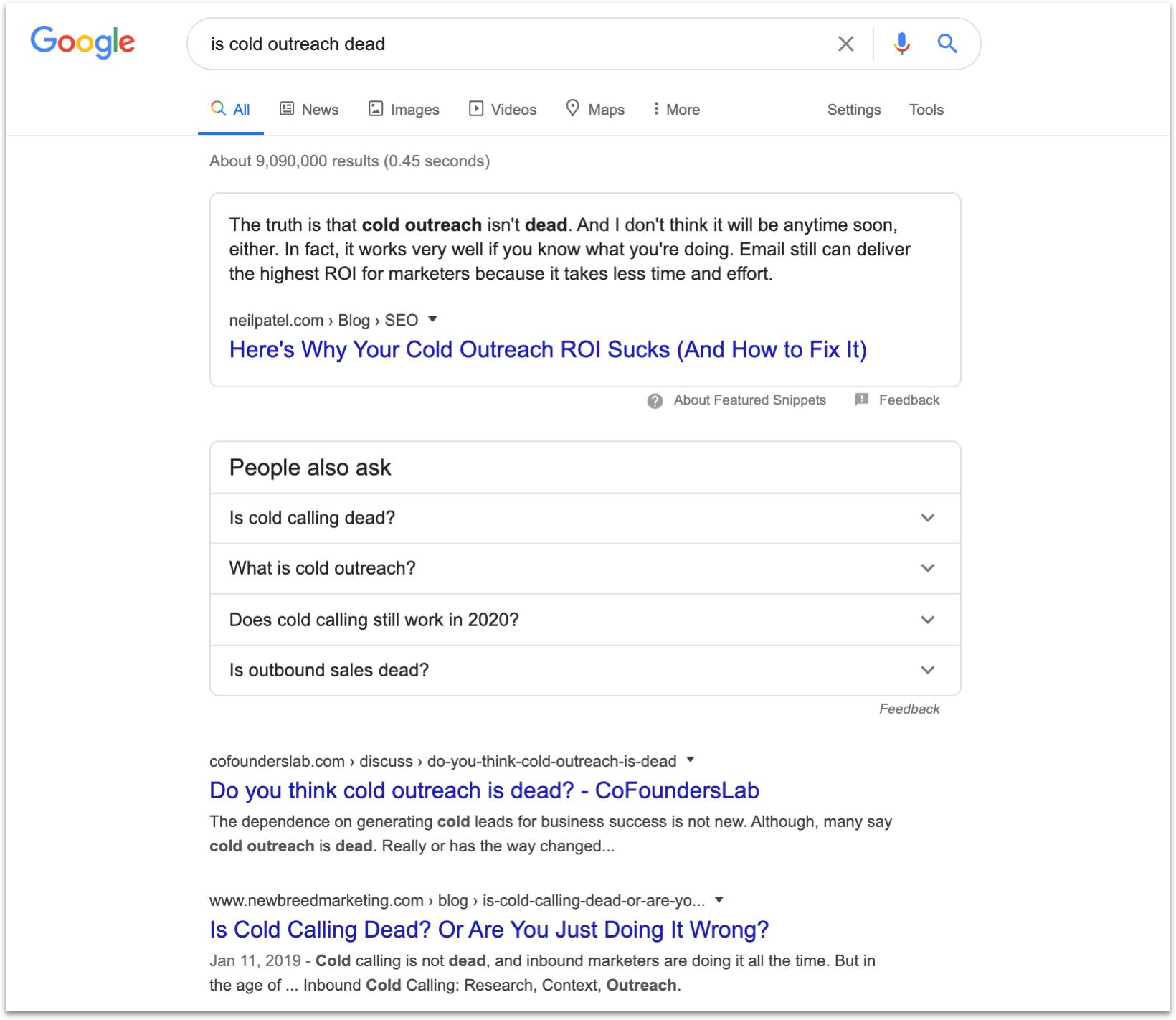In the image, a screenshot of a Google search results page is shown. At the top left, the Google logo is visible. Below it, the letters "G," "O," "O," "G," "L," and "E" spell out "Google" in a sequence. The search query typed is "Is cold outreach dead?" 

On the right side, there are icons for closing the search ('X'), activating voice search (a microphone), and initiating the search (a magnifying glass). The search results are categorized by tabs including "All," "News," "Images," "Videos," "Maps," "More," "Settings," and "Tools."

The page indicates approximately 9,090,000 results returned in 0.445 seconds. The excerpt from the first few search results reads: "The truth is that cold outreach isn't dead, and I don't think it will be any time soon either. In fact, it works very well if you know what you're doing. Email still can deliver the highest return on those markers because it takes less time and effort." The text continues to discuss topics like blog SEO and how to improve cold outreach ROI. 

There is also a section titled "People also ask," featuring questions like "Is cold calling dead?" "What is cold outreach?" "Does cold calling still work in 2020?" and "Is outbound sales dead?"

An article snippet from Co-Founders Lab states, "The dependence on generating cold leads for businesses is not new. Although many say cold outreach is dead, there are also exchanges debating it, with claims that 'cold calling is dead' and 'cold calling is not dead'. Inbound marketers are engaging in cold calling all the time. Despite advancements in digital marketing and changes in sales tactics, traditional cold outreach methods still hold relevance."

This is a comprehensive view of a Google search results page responding to the query "Is cold outreach dead?"